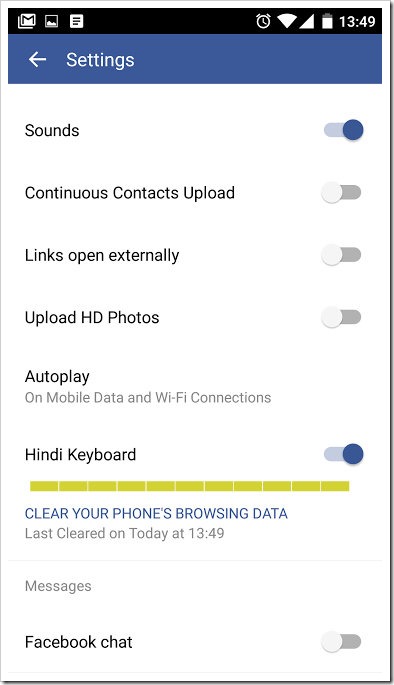This screenshot appears to be from a mobile device, specifically showcasing the settings menu of an application. The top portion of the screen features a black status bar typical of mobile devices, displaying standard icons such as the Gmail "M" icon and the Photos app icon on the left, alongside the battery icon, a clock reading "13:49," and a few additional icons on the right.

Beneath the status bar, a blue header with the word "Settings" in white text is prominently displayed, indicating that the user is within the settings menu of the app.

The options in the settings menu each have toggle switches and are listed in the following order:
1. **Sounds**: The toggle is blue and positioned to the right, indicating that this option is enabled.
2. **Continuous Contacts Upload**: The toggle is white and positioned to the left, indicating that this feature is disabled.
3. **Links Open Externally**: The toggle is likewise white and to the left, meaning it is turned off.
4. **Upload HD Photos**: Also toggled to the left and white, indicating this feature is disabled.
5. **Autoplay**: Accompanied by a Hindi keyboard option, this toggle is blue and positioned to the right, signifying it is active.
6. **Clear Your Phone Browsing Data**: A separate option not linked to a toggle switch but listed amongst the settings.
7. **Facebook Chat**: This toggle is white and to the right, suggesting it might be in an indeterminate state.

Overall, the settings menu is displayed against a clean white background, providing a clear and organized layout of each option and its current state.